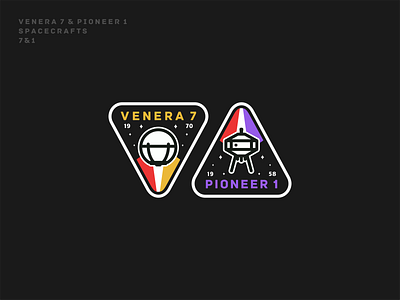The image features a stark black background with a nearly square layout, slightly wider than it is tall. At the top, in small, gray uppercase letters, it reads "VENERA 7 AND PIONEER 1 SPACECRAFTS." Central to the image are two adjacent rounded-off triangles, outlined in white. The triangle on the left has its base at the top, and inside it, "VENERA 7" is written in yellow letters with a white orb-like object beneath, detailed with red and yellow hues. Above the triangular emblem, "1970" is written in white, accompanied by small star-like details in the background. The right triangle points upward, with "PIONEER 1" inscribed in purple at the bottom and a red, white, and purple design at its peak. The orb within this triangle resembles a spacecraft. Similarly, "1958" is noted at the top, completing the celestial theme with more white stars scattered around.